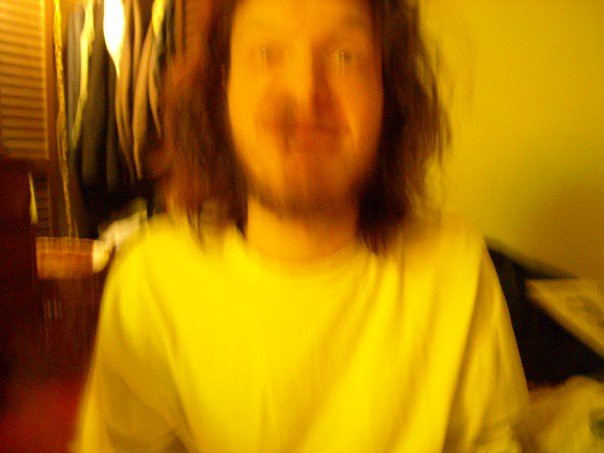In this blurry, out-of-focus image, a man with a neutral expression stares straight ahead. He is wearing a loose-fitting, long-sleeve yellow shirt. His long, scraggly brown hair frames his face, and he sports a thin mustache and beard. Behind him, a clothes cupboard filled with hanging garments or possibly a curtained window is visible. To his right, there is some periodical or printed material, with an indistinct pile of clothes below it. On the left side of the image, a wicker hamper is placed prominently in the center, while the upper left corner reveals part of a window blind.